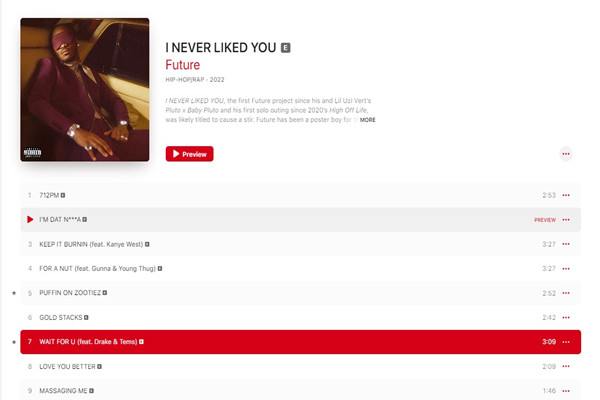Caption: 

The image displays a detailed track list for Future's album "I Never Liked You." At the top of the screen, the album's title is presented in bold black font with an "E" in a gray box next to it, denoting explicit content. The album title is highlighted in red alongside the genre tags "hip hop" and "rap," with the release year "2022." This album marks Future's first solo project since 2020’s "High Off Life" and follows his collaboration with Lil Uzi Vert on "Pluto x Baby Pluto." 

In the left section of the image, there is a photograph of Future dressed in a striking purple suit complemented by silver jewelry. He wears a purple eye mask and appears to be lounging in the backseat of a car, exuding a relaxed yet stylish demeanor.

Below, the track list is clearly outlined. The currently playing or previewed track, "I'm That N***a," is indicated next to the time "7:12 PM." The list continues with:
1. 7:12 PM
2. I'm That N***a
3. Keep It Burnin (feat. Kanye West)
4. For A Nut (feat. Gunna and Young Thug)
5. Puffin on Zootiez
6. Gold Stacks
7. Wait For U (feat. Drake) - Highlighted in red
8. Love You Better
9. Massaging Me

A red "preview" button is situated below the track list, inviting listeners to sample the album's content.